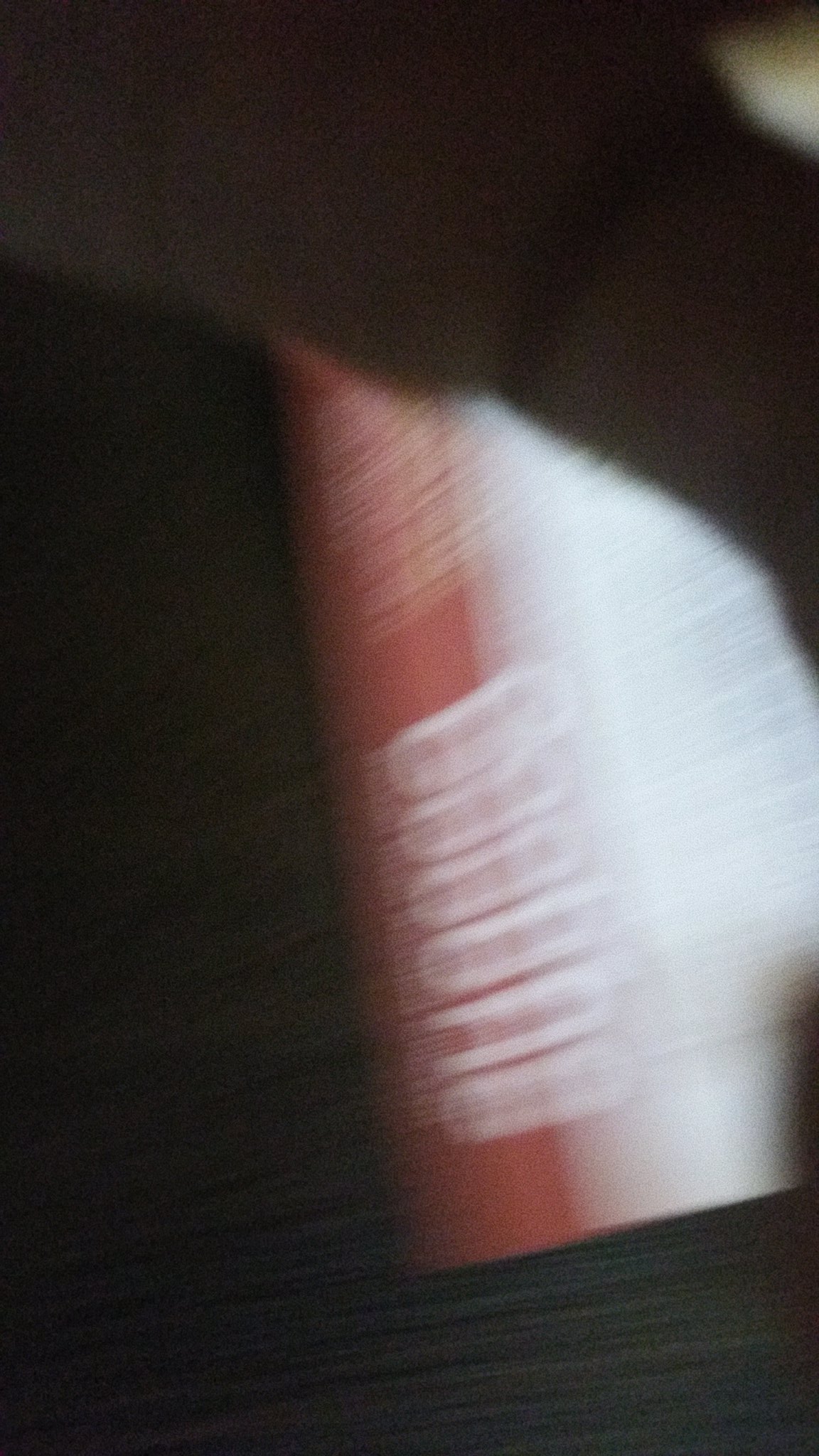The image is extremely blurry and difficult to decipher, with the background appearing predominantly black. In the lower left corner, extending somewhat to the center bottom, there's a distinct black shape. The center of the image features a red and white object; the red section is at the bottom and has some indistinct white writing. At the top, a long brown shape extends over this red and white object, giving the impression of depth or obstruction. The entire image seems to be in motion, further blurring potential text and fine details. The presence of colors like red, white, black, brown, and gray is noticeable, and there seems to be an interplay of shadows and light, possibly indicating another object like a hand or arm partially obstructing the view of the central red and white figure.